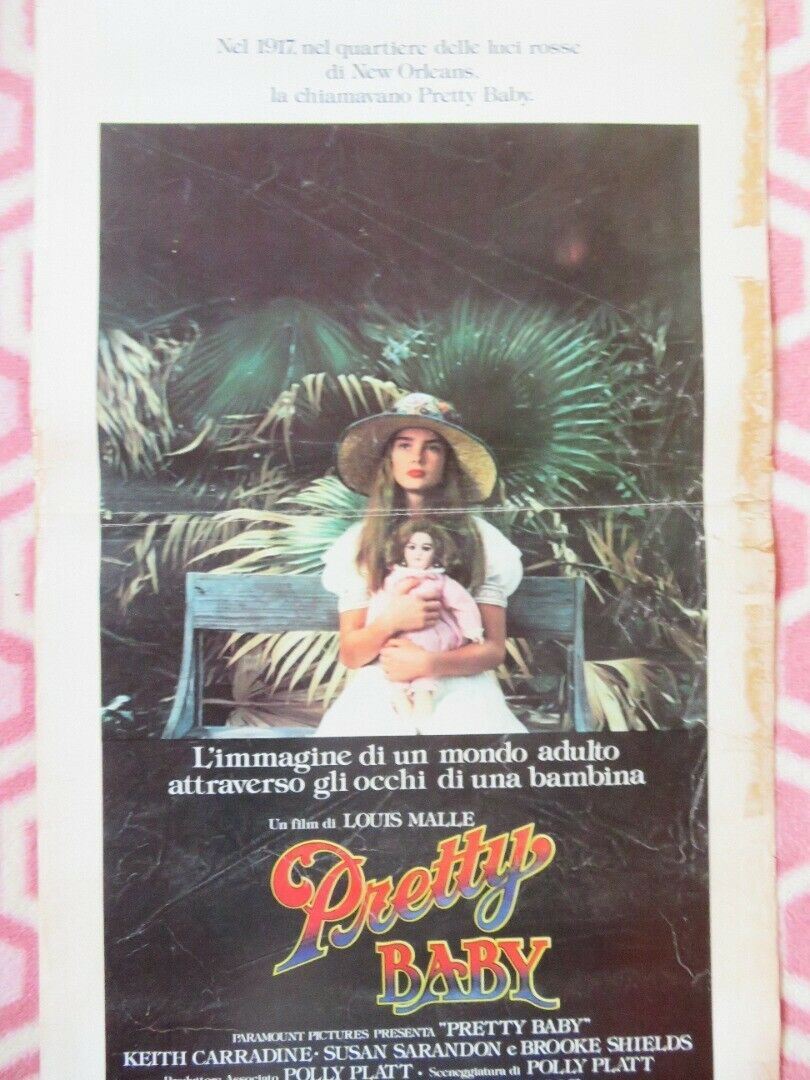This is a vintage movie poster for the film "Pretty Baby" presented by Paramount Pictures. The poster primarily features the young actress Brooke Shields, who is seated on a blue bench holding a doll dressed in pink with brown hair. Brooke Shields, identifiable by her brown hair, is wearing a white dress and a sun hat. She is surrounded by lush, tropical plants. The text on the poster includes the title "Pretty Baby" prominently displayed in red and purple, and additional credits listing the stars Keith Carradine, Susan Sarandon, and Brooke Shields. The text is in a mix of languages, with some parts in French and possibly Italian, including phrases like "Le film de Louis Mal" and other promotional details. The right side of the paper looks worn and stained, adding a vintage feel to the overall image.